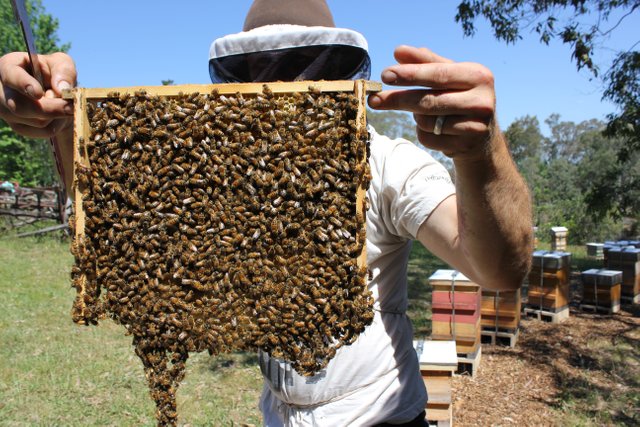The image captures a beekeeper, identifiable by his protective gear, comprising a white t-shirt and a hat with black netting covering his face. He is showcasing a wooden frame filled with busy honeybees to the camera, likely a component of a beehive. His left hand, adorned with a silver wedding ring, and his right hand grip the frame tightly. Around his waist are visible ties, possibly part of his beekeeping outfit. The frame, small and square with a yellowish wooden hue, swarms with an estimated 500-1000 bees forming dense clusters on the combs. The beekeeper stands at a slight diagonal angle under a bright sky, amidst an array of beekeeping equipment and nature. The background reveals a mixture of grass, trees, bushes, and several beehives, showcasing the prolific environment where his craft thrives.